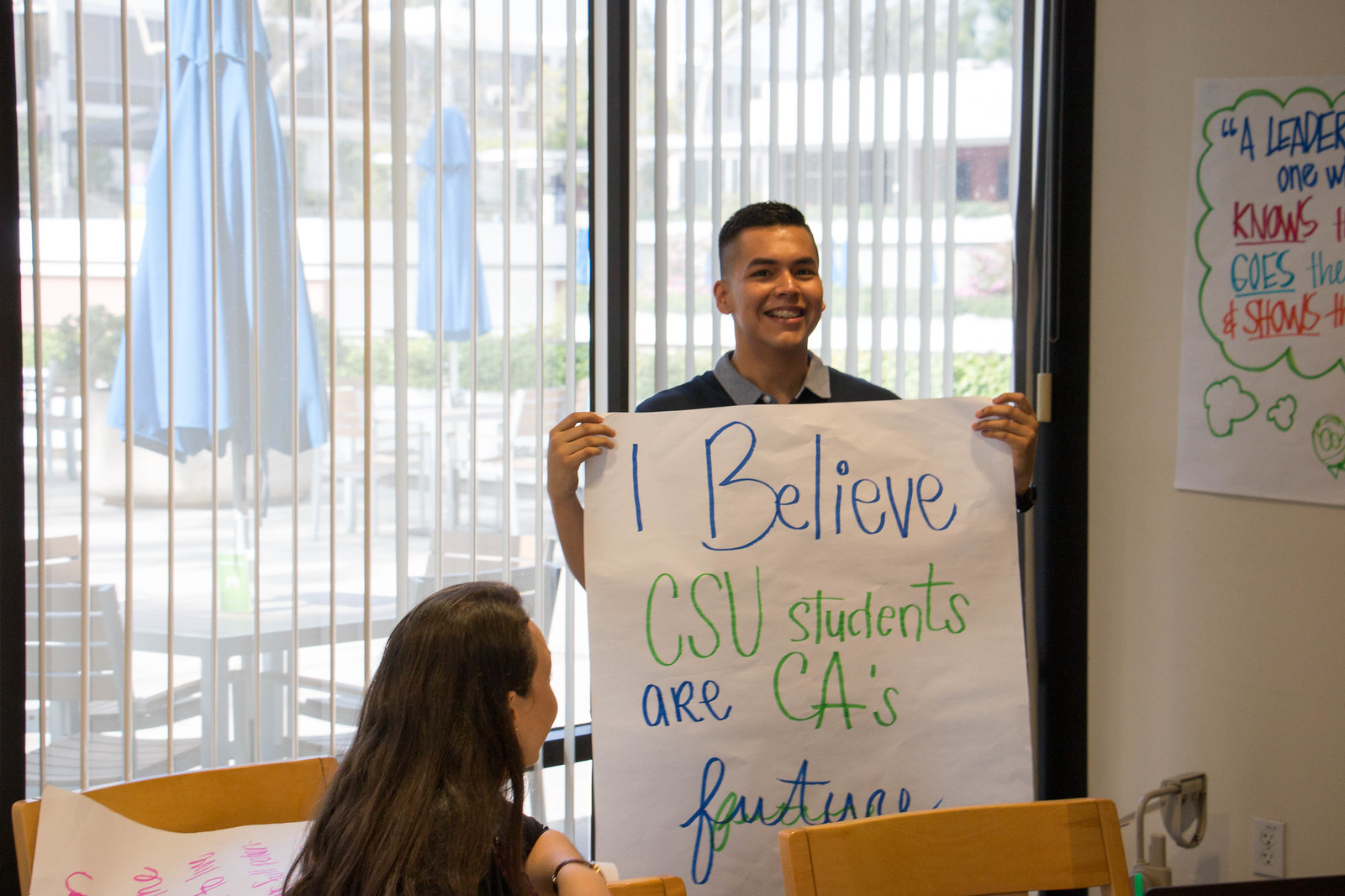In this detailed image, we see a young man with slightly tanned skin, possibly of Hispanic or Southeast Asian descent, standing in the center of a room. He has dark brown hair, shaved on the sides and short on top, and is smiling while looking at the camera. He is holding a large white poster board that covers his torso, on which the message "I believe CSU students are CA's future" is written in blue and green marker. The poster spans from his shoulders down to the edge of the frame, hiding his body.

To the left and slightly in front of him, there is a seated woman with long brown hair wearing a black shirt. Only the back of her head and part of her arm are visible. The setting appears to be a classroom or similar indoor environment, characterized by white walls, vertical floor-to-ceiling windows with blinds, and various tables and chairs.

On the right wall, there's a partially visible poster with motivational text that reads "A leader knows, goes, shows," with the rest obscured. An electrical outlet is visible at the bottom of this wall. Through the windows, one can see an outdoor area with tables, umbrellas, and surrounding chairs, indicating a cafeteria courtyard. Also visible are green plants growing outside. The scene is brightly colored with various hues including tan, white, green, blue, red, light blue, orange, and pink, suggesting it is taken in the middle of the day.